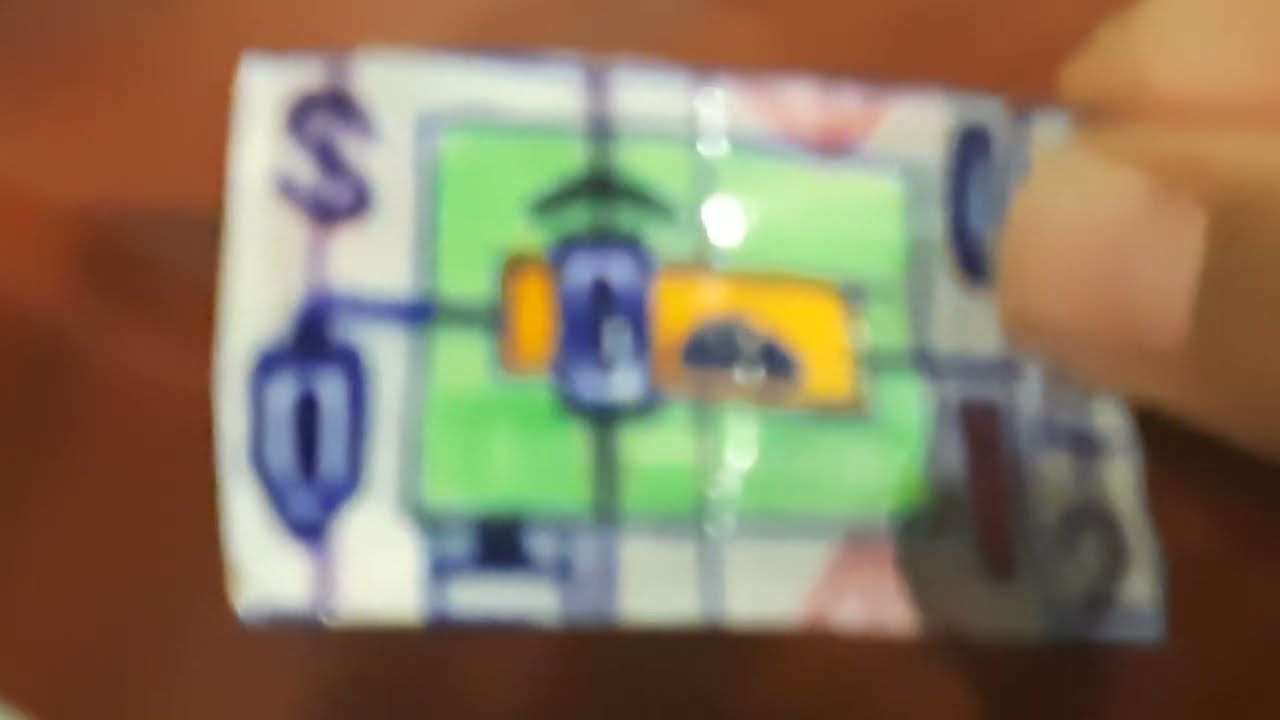This horizontal rectangular image is notably blurry, especially around its borders, which are predominantly brown with some darker brown patches. At the center of the image, a person's hand emerges from the right side, displaying a thumb and index finger that are clutching an object. This object, resembling a horizontally aligned card or folded piece of paper, is approximately the size of a standard card.

Despite the blurriness, some details on the card can be discerned. The card has a predominantly white background, adorned with various illustrations and text. Notably, there is a blue "S" located on the upper left side and possibly a number "3" on the lower right. The central part of the card features a green square outlined in blue, with a yellow rectangle inside. Vertically, there are lines dividing sections, and horizontally too, dividing the space further. Inside the yellow rectangle, there appears to be an "O" on the left and a black arrow pointing upwards. Other images and letters, including an "O" at the bottom right and a tree-like design, are not clearly visible due to the blurriness.

Overall, the image's defining characteristics are its significant blur, the hand holding the card, and the mix of white, blue, yellow, and green colors on the card, combined with unclear illustrations and text.